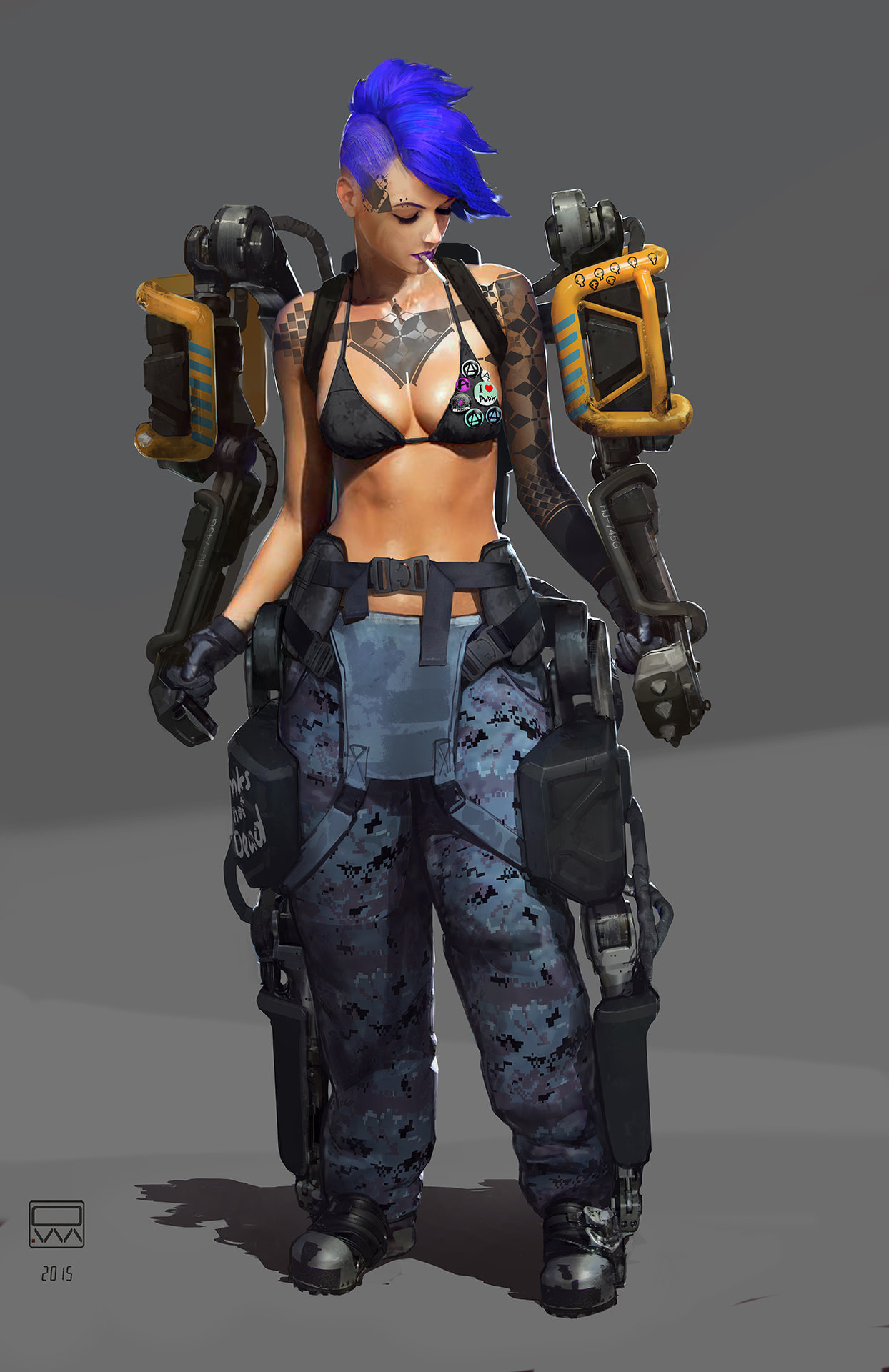In this image, set against a dark gray and light gray background, a distinctive game character stands out. The character features short blue hair, meticulously shaved on the left side and stylishly combed over to the right. She is clad in a black bikini top, revealing her midriff and toned torso. Her right arm is adorned with a black and yellow device that resembles a powerful weapon.

Tattoo art spans across her chest, starting from her shoulder and extending to the other shoulder, adding an element of fierce elegance. Around her waist, she sports a tactical belt laden with various weapons, highlighting her readiness for battle. She wears a pair of overalls, though the front bib is casually left undone, giving off a relaxed yet prepared vibe. The overalls themselves are a grayish-blue color, speckled with black.

Her ensemble is completed with sturdy black boots, and additional weapons are strapped along both sides of her legs, emphasizing her combat-ready stance. The intricate details and the assortment of weaponry suggest she is a formidable character from an action-oriented game.